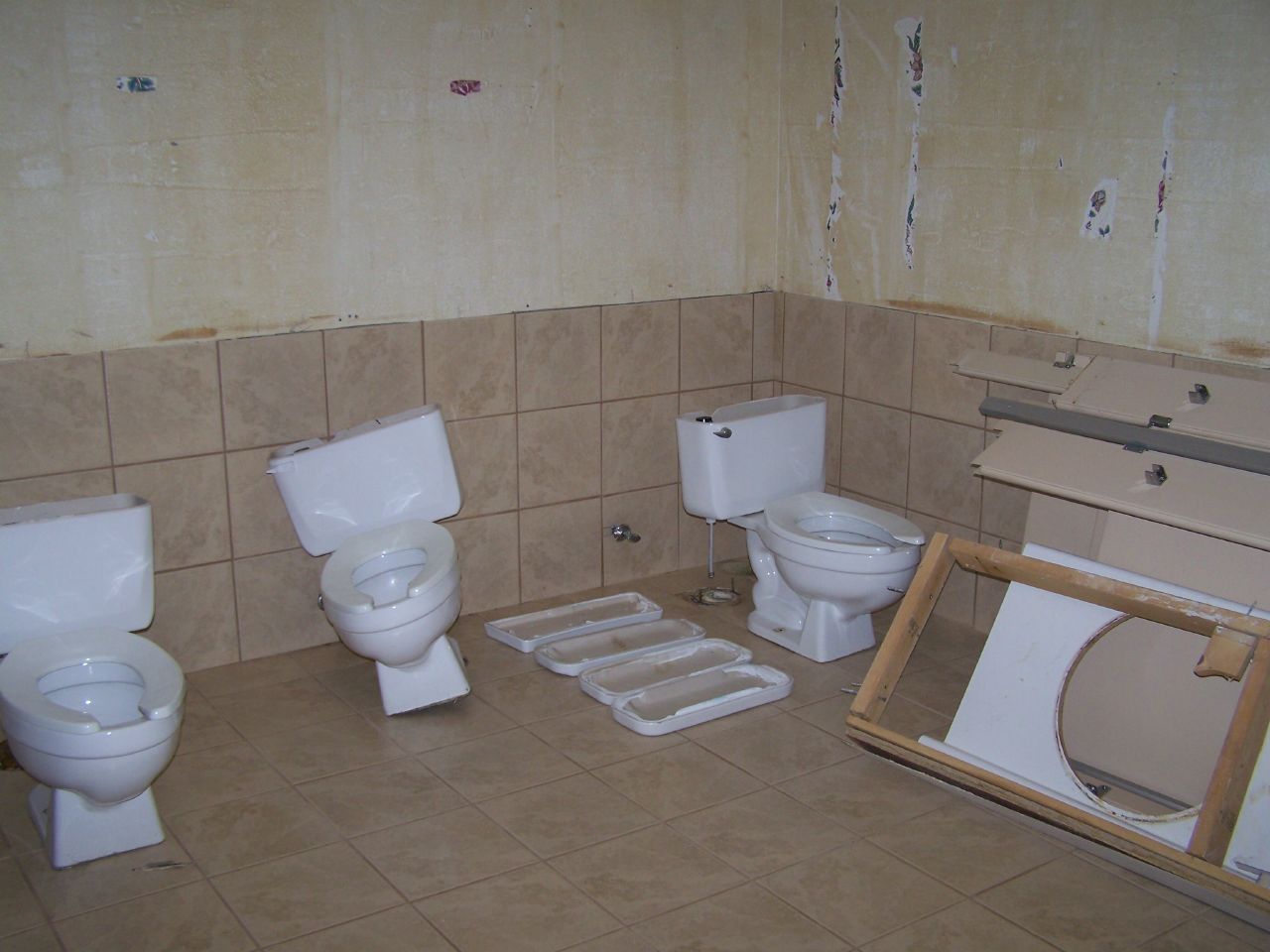The image is a detailed color photograph of a public restroom undergoing extensive remodeling. The tiled walls are covered with large beige tiles, possibly 18 inches by 18 inches, extending about three feet up the wall. Above this, the upper part of the walls is in disrepair, appearing white streaked with yellow stains, likely the remnants of removed wallpaper or old gluing material, giving it a dirty appearance.

In the center and left part of the room, three white porcelain toilets are visible, none of which are properly mounted. One toilet leans awkwardly against the wall at an angle, while the other two are more or less upright but still not connected to any plumbing. Additionally, there are four toilet tank lids lying inverted on the floor, indicating the presence of one more toilet not visible in the photograph.

Piled against the right wall are dismantled stall partitions in a beige color, typical of public restroom dividers, indicating that the stall walls have been completely removed. There is also a white board with a circular cutout and some metal framework, possibly part of a sink setup or other construction materials, adding to the sense of ongoing renovation.

The floor is uniformly tiled with the same beige tiles found on the lower walls, which appear to be in decent condition and likely to be retained after remodeling. Cardboard boxes and other construction debris are scattered throughout, further illustrating the state of transformation this bathroom is undergoing.